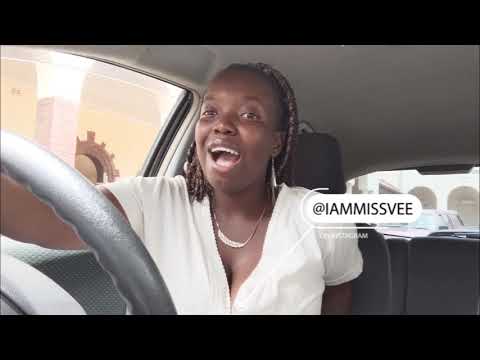In this color photograph taken from the dashboard inside a vehicle, an African woman with dark skin and brown braided hair is seen sitting in the driver's seat on the right side of the car, indicating that this might be in Europe or Africa. She appears happy, smiling or possibly talking with her mouth wide open. The woman is dressed in a white short-sleeved shirt, accessorized with a gold necklace and gold earrings. The interior of the car is predominantly gray, including the upholstery and the headrest. To the left side of the image, the car window reveals a tan or yellow wall, possibly a side of a building, with a circular brown item attached to it. On the right side of the image, there is a white tag saying "I am Miss VEE," suggesting it could be an advertisement for her website. The exterior background also shows arches from an Adobe-like building. Additional cars can be seen behind her, contributing to the bustling small town atmosphere.